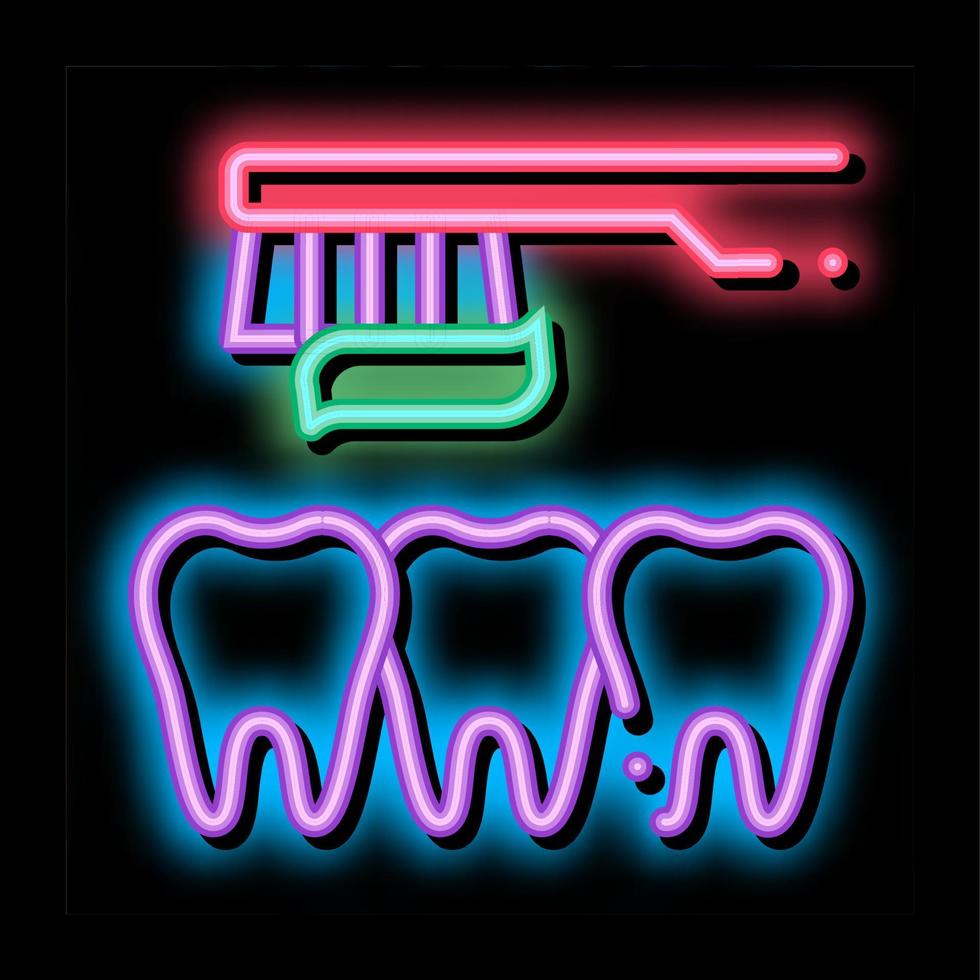This visually striking neon art piece features a black background that sets the stage for a vivid, contemporary design. Dominating the upper section, a bright red neon toothbrush handle extends vibrant purple bristles downward. A streak of lime green neon simulates a strip of toothpaste, making contact with the bristles. Below, three large tooth shapes, outlined in purple and shaded with dark teal blue, display a modern, stylized aesthetic. The teeth have dark centers, evoking the appearance of cavities, while the rightmost tooth shows a distinct break highlighted by a pink dot. This composition captures the dynamic interaction of the toothbrush with the teeth, enhanced by the vivid illuminations of neon lights.